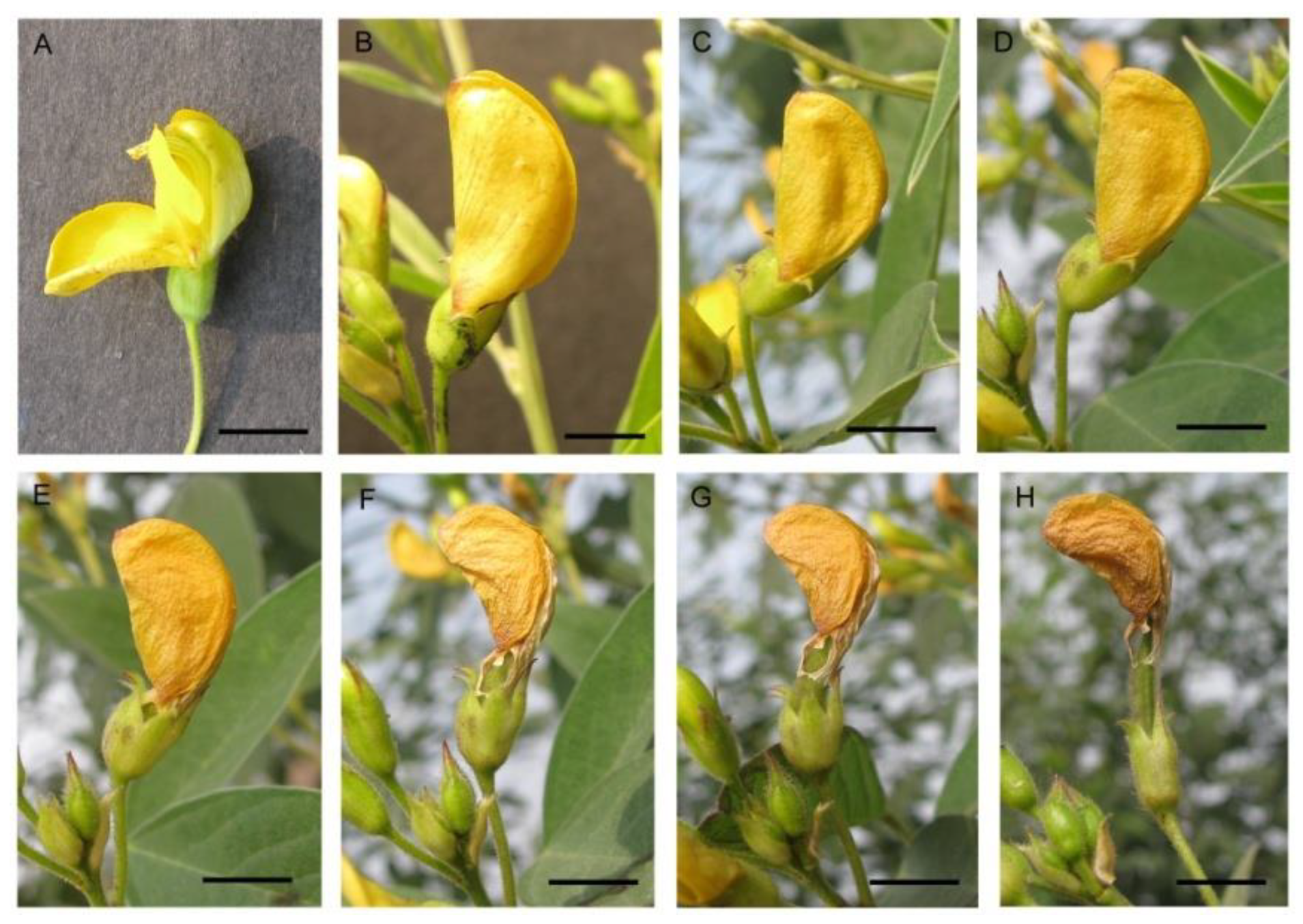The image is a series of eight photographs labeled A through H, arranged in a two-by-four grid, depicting the stages of a yellow flower's life cycle from vibrant bloom to complete decay. In the first image (A), the flower is fully open, displaying vibrant yellow petals and healthy green leaves. As we progress to image B, the flower begins to close, with the outer petals showing hints of tan. By image C, a darker tan color starts to dominate, and the petals begin to lose their vitality. In image D, the tan intensifies and the petals show initial signs of shriveling. Moving to image E, the flower appears more orange and is starting to separate from the green stem, exhibiting significant dryness. By image F, the flower has major wrinkles and is significantly decayed, with parts of it coming apart. Image G shows the flower in an even darker shade of brown, further detached and eroded. Finally, in image H, the flower is completely shriveled, unrecognizable, and almost totally disconnected from the stem, resembling a peanut in a shell, marking the end of its life cycle.